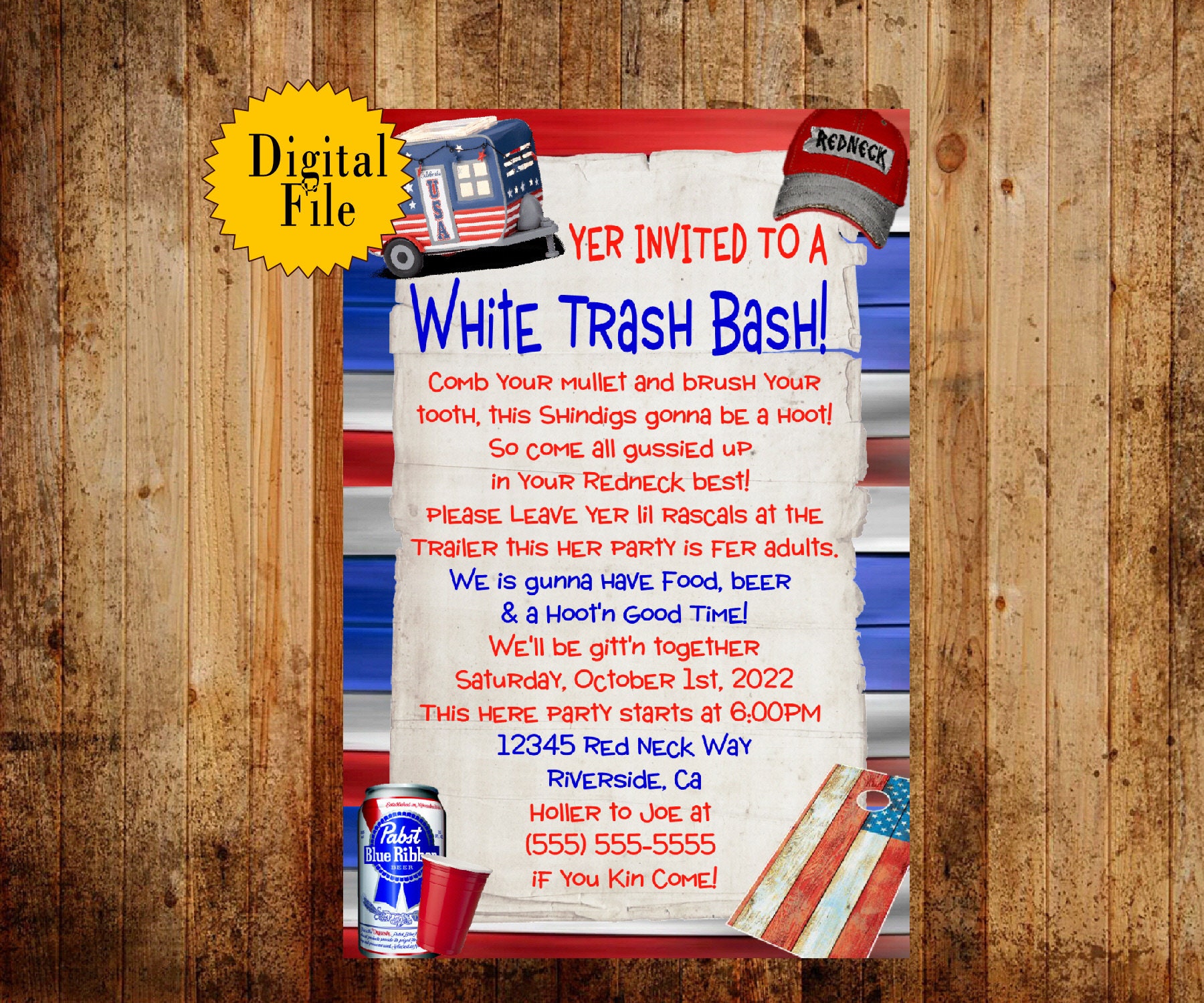This photo displays a digital invitation flyer set against an aged, dirty wooden background composed of weathered boards. The colorful flyer, designed in red, white, and blue hues, prominently invites recipients to a "White Trash Bash." The invitation humorously urges guests to "Comb your mullet and brush your tooth," promising a lively event with "food, beer, and a hootin' good time." It specifies the party is adult-only, advising attendees to “leave your little rascals at the trailer" and to dress in their "redneck best." The bash is scheduled for Saturday, October 1st, 2022, starting at 6 p.m., taking place at 1234 Redneck Way, Riverside, California. Attendees are requested to RSVP to Joe at 555-555-555. Surrounding the central text are illustrations including a camper trailer, a redneck hat, a Pabst Blue Ribbon beer can, a red solo cup, and a bean bag toss game, all reinforcing the playful, rustic theme of the event.